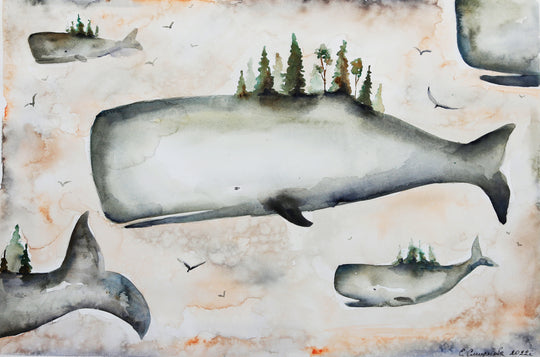This abstract painting depicts a surreal scene with multiple whales of varying sizes, primarily rendered in shades of white and gray, swimming amidst a fluid, bleeding watercolor background. Central to the composition, the largest whale draws immediate attention with its distinctive features—thin mouth opening, small eyes, and surreal trees growing from its back. The other whales, including a smaller one in the lower right and another partially visible in the lower left, share this bizarre characteristic with trees sprouting from them as well. A few birds can be seen flying around, adding to the whimsical yet enigmatic nature of the artwork. The overall theme interweaves elements of marine life and terrestrial flora, creating a unique, symbolic narrative. Although there is some text or markings in the lower right, it is illegible, potentially indicating the artist's signature or date. The color palette subtly incorporates hints of orange and light blue, complementing the main grayscale depiction of the whales and their unusual adornments.